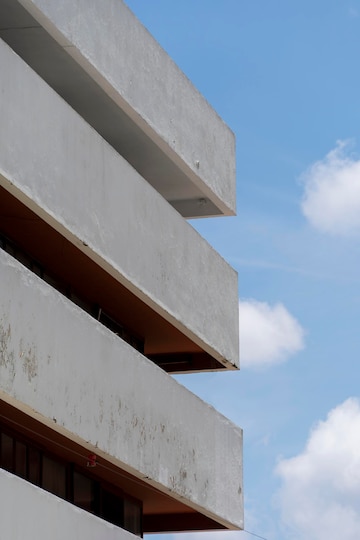The image depicts a daytime scene with a light blue sky adorned with a few puffy white clouds on the right side. Dominating the left side of the photo is a multi-level, brutalist-style concrete structure that appears to be a parking garage. The building features visible overhangs and ledges, with three prominent levels. The middle two levels are characterized by an orange, rusty hue, suggesting wear, while the top level showcases the raw gray concrete. Additionally, there are some small hanging lights and windows framed in black with curtains inside.